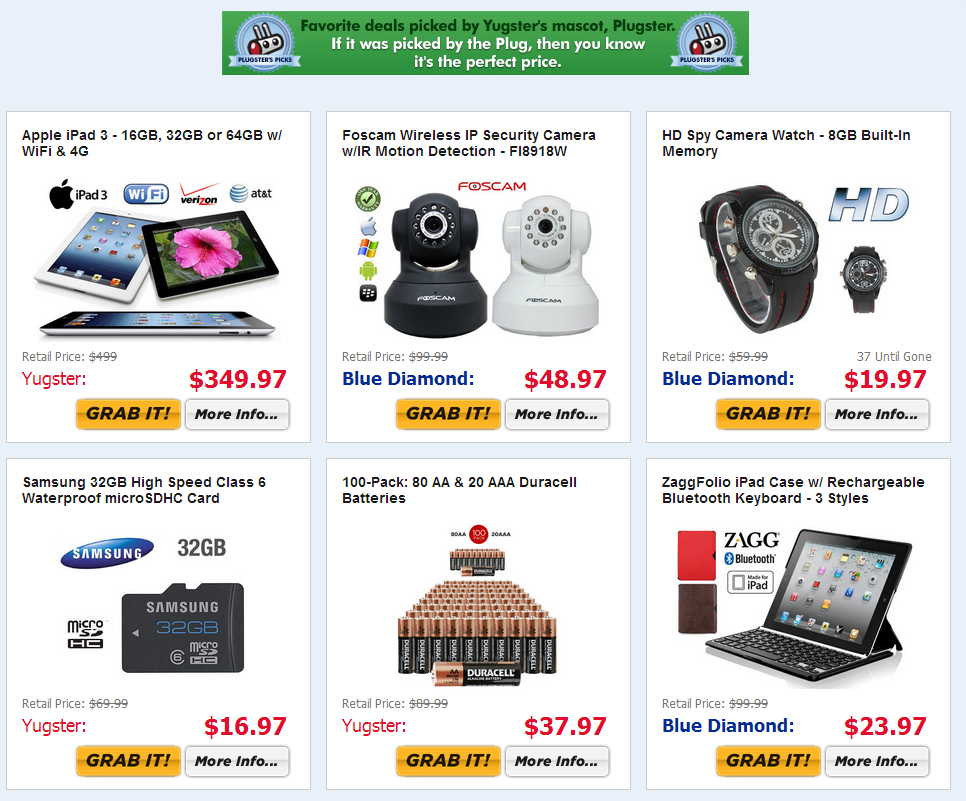This is a detailed and organized caption for the described image:

---

**Favorite Deals Picked by Youngster's Mascot, Plugster**

The flyer features a prominent bold green banner at the top, announcing "Favorite Deals Picked by Youngster's Mascot, Plugster" with blue stamps on either side, each containing a little face inside a plug, symbolizing Plugster.

The advertisement presents six carefully selected items in a grid layout, three items across and two items down:

1. **Youngster Product** - Highlighting the brand's unique offering.
2. **Apple iPad 3** - A sleek and intuitive tablet for all your digital needs.
3. **Foscam Wireless IP Security Camera** - Ensuring home security with advanced monitoring capabilities.
4. **HD Spy Camera Watch** - Combining style with discrete surveillance.
5. **Samsung 32GB High Speed Class 6 Waterproof Micro SDHC Card** - Durable and efficient storage solution for various devices.
6. **100 Pack Duracell AA and 20 AAA Batteries** - Reliable power for all your gadgets.

Additionally, the flyer features the **Zagfolio iPad Case with Rechargeable Bluetooth Keyboard**, available in three stylish designs to enhance your iPad experience.

Pricing is prominently displayed as "Youngster Price" with a call-to-action button labeled "Grab It" for further details on each item.